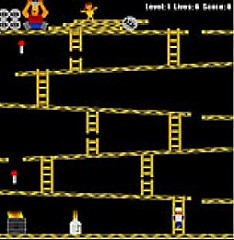This is a detailed scene from an 80s retro-style video game with a black, square background. It features six platforms, each interconnected by yellow ladders, some of which are broken apart, making navigation challenging. The very top platform holds a larger man clad in blue pants and a red shirt, seemingly sitting, and next to him stands a smaller character dressed in yellow. The man appears to be throwing a circular object. On the left side of the screen, there are two items characterized by long white rectangular bases and red circular tops. At the bottom platform, there is a square emitting an orange hue and a large bottle. A smaller figure, wearing blue pants and a white top, is seen climbing the first ladder. In the upper left corner of the screen, there are two white circles in a vertical alignment above another pair. To their right is an orange-yellow rounded character with black vertical lines for eyes and a red mouth. Additionally, there is yellow and brown checkered road-like squares diagonally bisecting the screen from this character. The game's interface also includes undecipherable white text and digits indicating the level in the upper right-hand corner.